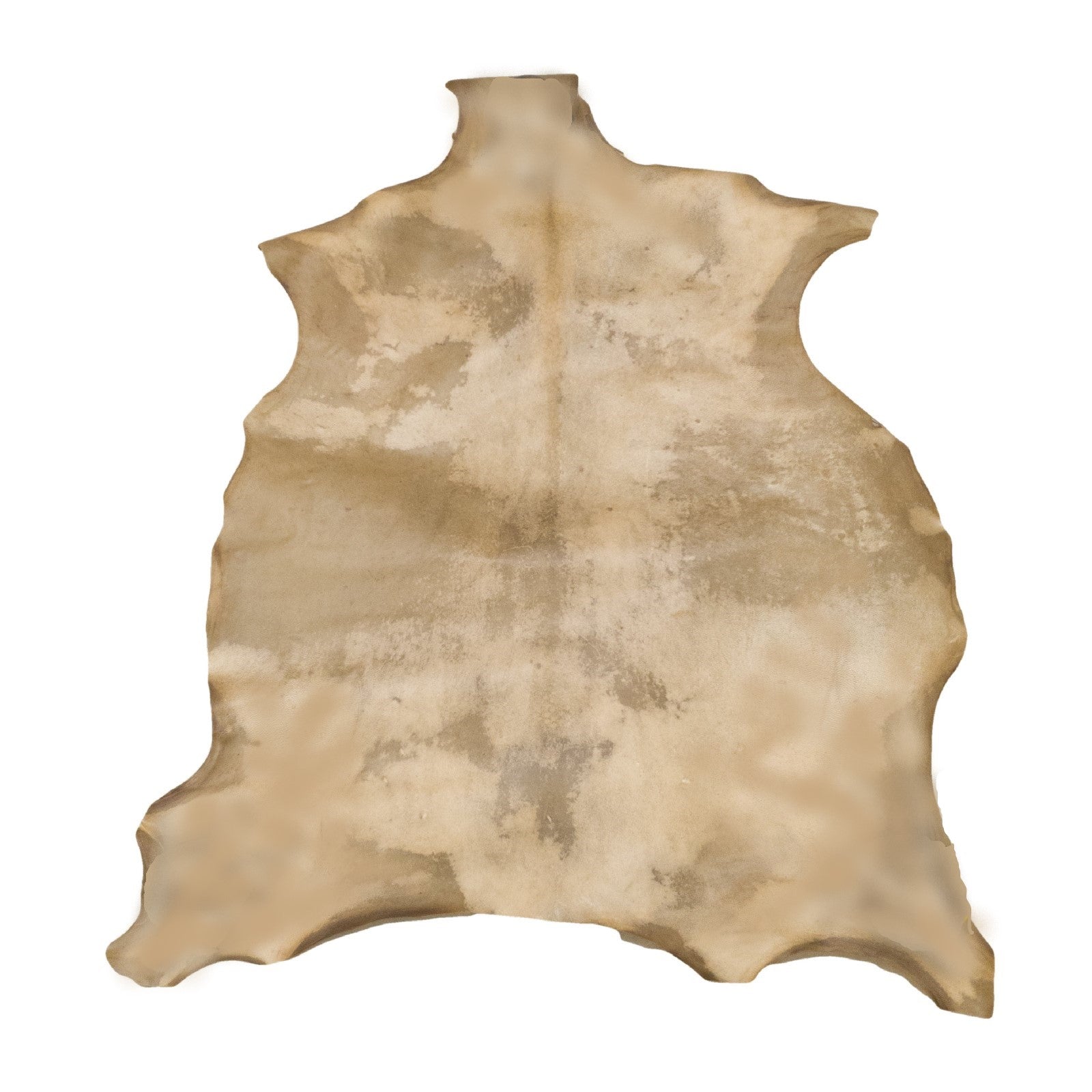This is a highly detailed image of an animal hide, possibly that of a goat or bear, laid flat on a white background as if for a product shot. The hide exhibits a light brown or tan color with mottled shades of beige and brown, featuring some dark striations that could indicate the spine area. The edges of the pelt are scalloped, and the shape hints at visible anatomical features: the top appears to be where the neck was cut, while the left and right sides resemble parts of two arms. At the bottom, a pair of sections suggests where the feet of the animal might have been. The hide itself has been stretched out, possibly intended as a rug or wall hanging.